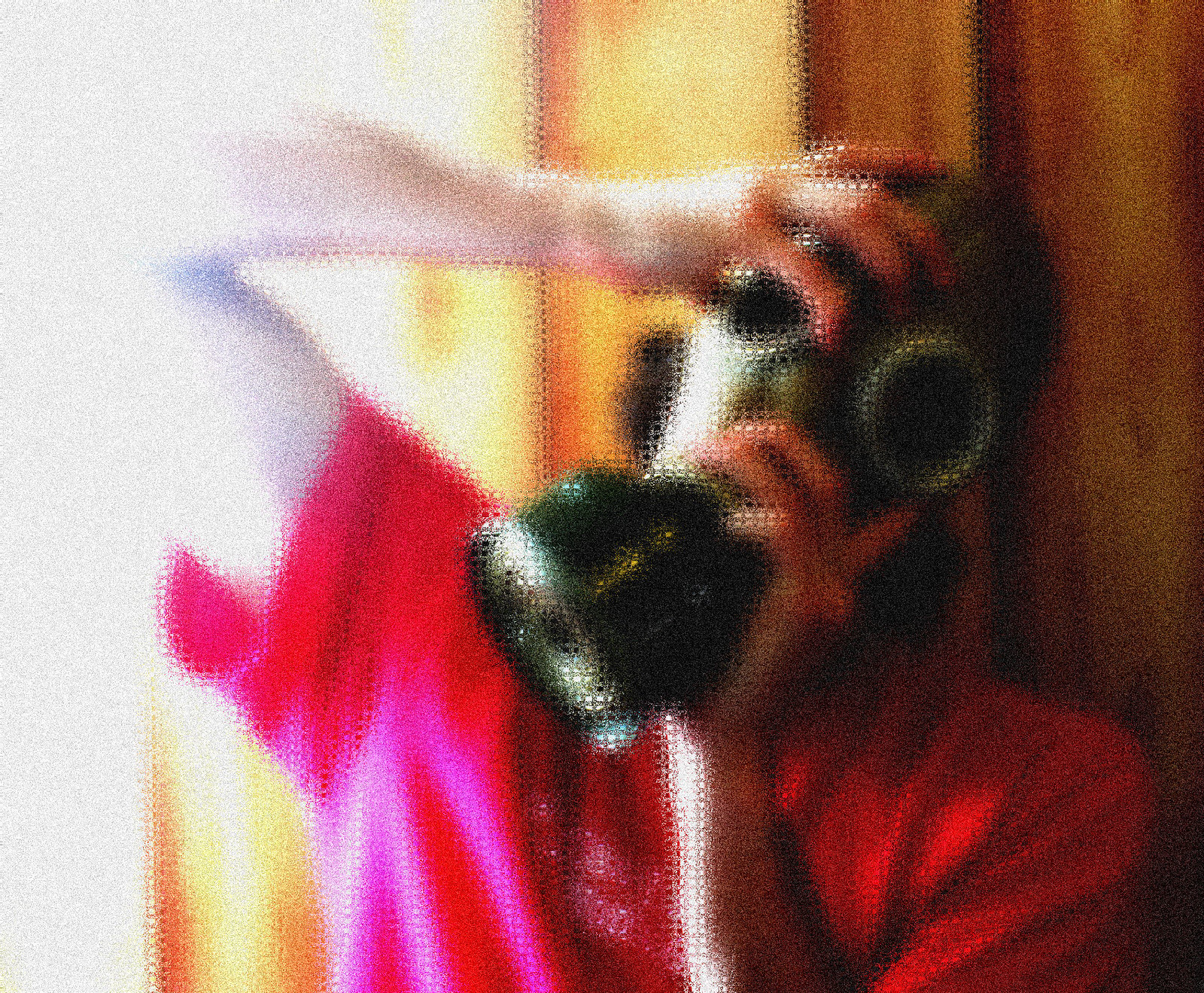The image depicts an indoor setting with a very blurry and pixelated quality, giving it a distorted appearance. A white man is centrally positioned, wearing a red t-shirt and holding an old-style World War I or World War II gas mask over a canister on his face. The gas mask features dark lenses, obscuring his facial features. He is grasping the mask with both hands, one positioned on the canister and the other stretched above and touching the top of the mask area. The background consists of a brown wall with what appears to be wood paneling, possibly a door, on the left-hand side. This section of the wall is illuminated by a light, casting a yellowish tint, while the very left edge of the image fades into white.